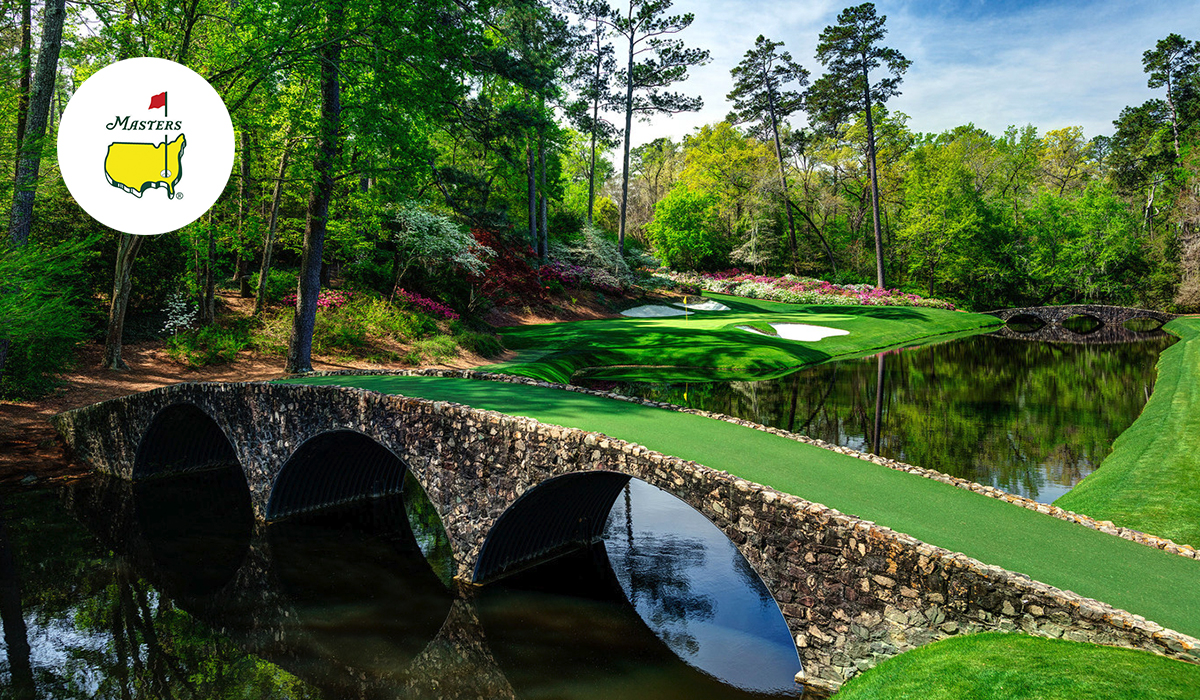This photo depicts a meticulously manicured landscape of a prestigious golf course, identifiable by the Masters logo, which features the outline of the United States with a flag, prominently displayed in a white circle on the left. The lush green turf blankets the course, extending to a distant hole dotted with sand traps. Two elegant footbridges span a sparkling, mirror-like creek, their stone arches reflected in the water's pristine surface. These bridges have thick green grass on top, harmonizing with the surrounding vegetation. The backdrop showcases a vibrant forest of green trees against a backdrop of blue skies with hazy white clouds, adding to the serene and well-kept appearance of the scene.